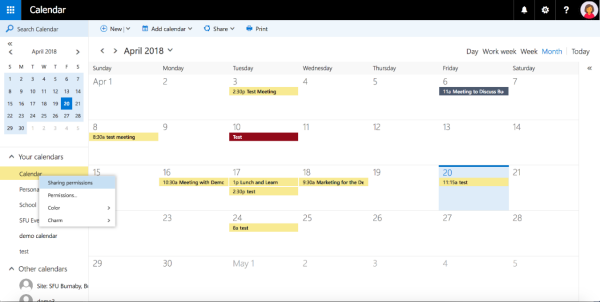In this image, a calendar application interface is displayed in a zoomed-out view. At the top left corner, there is a small blue square containing nine dots. Next to this square, "Calendar" is written in white text. On the upper right corner, there are icons for notifications, help (depicted by a question mark), and a user profile picture against a black background.

Below these icons, there is a "Search Calendar" bar, followed by four categories labeled to its right. The main section shows the calendar for April 2018. Among the dates, only April 20th is selected and highlighted in blue, while all other days are shaded in gray.

Beneath the calendar, there is a section titled "Your Calendars" with five categories listed. Following this, there is a section titled "Other Calendars" containing two categories. To the right side of the calendar, the month and year "April 2018" is displayed again, above a list of events noted with a variety of highlights: many are marked in a yellowish-gold color, one in dark red, and one in blue. The 20th of April, in particular, has a gray square highlighting the events or plans for that day.

At the top right corner of the interface, there are five additional categories with one highlighted in blue. Alongside, the word "Today" is visible near a very thin horizontal line running at the bottom edge of the image.